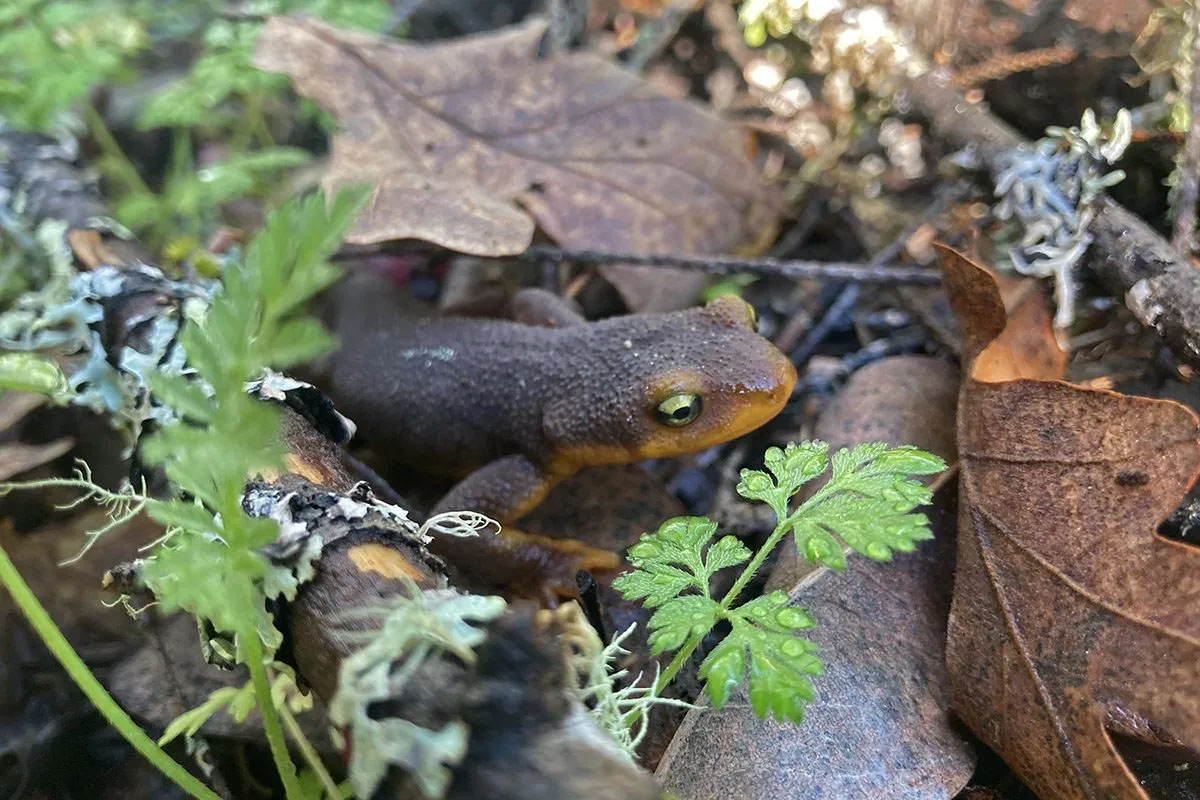The photograph captures a close-up view of a small salamander on a forest floor, blending remarkably well with its surroundings. The scene looks earthy and autumnal, with dark brown, dry leaves, twigs, and patches of green weeds scattered around. The salamander is at the center of the image, partially emerging from beneath a dead twig on the left side. Its coloration is a mix of dark brown on the top and a lighter, tan brown or yellowy orange underneath. The creature is crawling upwards and outwards towards the right, its slender right leg extended and bent as if grasping something beneath it. Its alert eyes are a striking green with dark black pupils. The detailed focus of the image emphasizes the natural camouflage of the salamander against the forest floor, while the slightly blurred background enhances the prominence of the small amphibian.